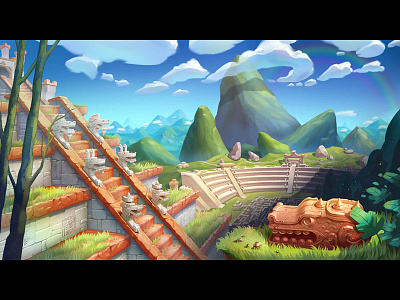This still image from a cartoon or animated video game depicts an ancient temple set amidst lush, vibrant mountains. The temple, built from white cinder blocks, features grand terracotta-colored stairs leading up to multiple levels, each adorned with green grassy terraces. Prominently in the mid-ground stands a large terracotta-colored statue of an alligator head perched on a grassy island. Flanking the staircase are statues resembling dragon heads or lizards. The imposing structure sits under a blue sky filled with white clouds, eight in total, three large and five small. In the background, an open-air arena blends seamlessly into the base of towering green mountains, adding a sense of depth to the scene. Additionally, a leafless tree occupies the left foreground, contributing to the picturesque and detailed setting. This vibrant image, capturing the interplay of nature and ancient architecture, showcases a distinct cartoony art style with vivid colors and intricate details.